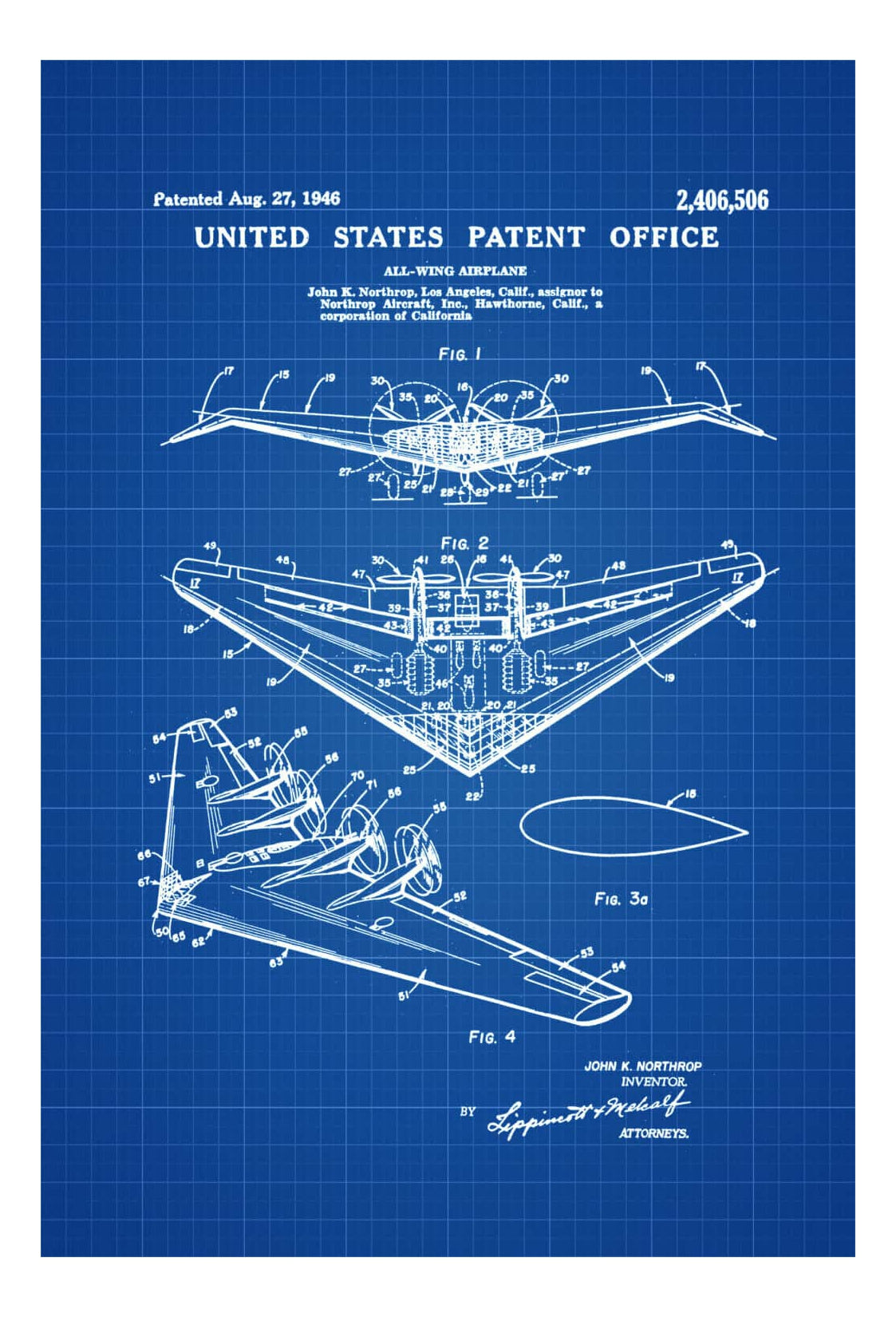This image is a detailed blueprint from the United States Patent Office, representing a patent for an all-wing airplane, primarily known as the Northrop Grumman flying wing, patented on August 27, 1946, with the patent number 2,406,506. The background is a royal blue graph paper with white grid lines. At the top, in white text, it states: "Patented August 27, 1946, 2,406,506, United States Patent Office, All-Wing Airplane, John K. Northrop, Los Angeles, Calif., Assigner to Northrop Aircraft, Inc., Hawthorne, Calif., a corporation of California." Beneath this heading, the blueprint displays four distinct figures illustrating various views and details of the aircraft. These views include a front view, a top view, and a three-quarter view, all depicted with sharp white lines. The aircraft features a distinctive boomerang shape with four propellers located at the rear. The illustrations are annotated with numbers and labels denoting different parts and measurements. At the bottom of the blueprint, it reads: "John K. Northrop, Inventor," accompanied by an illegible signature and the word "Attorneys." This patent blueprint showcases a comprehensive visual and textual description of the innovative all-wing aircraft design by John K. Northrop.